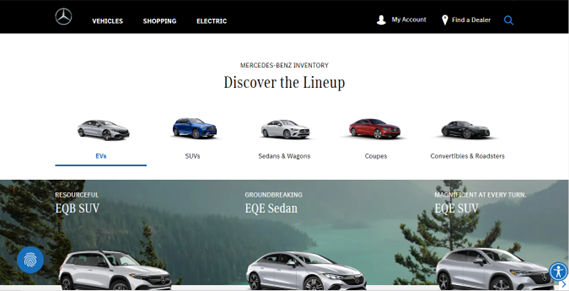In this image, a meticulously organized lineup of cars is displayed against a scenic backdrop, illustrating a range of Mercedes-Benz models. The lineup starts with a white car, followed by a blue car, another white car, a striking red car, a sleek black car, and finally four more white cars. Notably, these include electric models such as the EQB SUV, EQE sedan, and EDV SUV.

The picturesque background features two lush green trees and a serene body of water, under overcast gray skies. A verdant hill, tinged with patches of gray, adds depth to the scenery. 

At the top of the image, there is a black banner with white writing, while the bottom part of the image features a contrasting white background with black writing. Each car model is accompanied by a corresponding picture, adding a visual cue alongside its name.